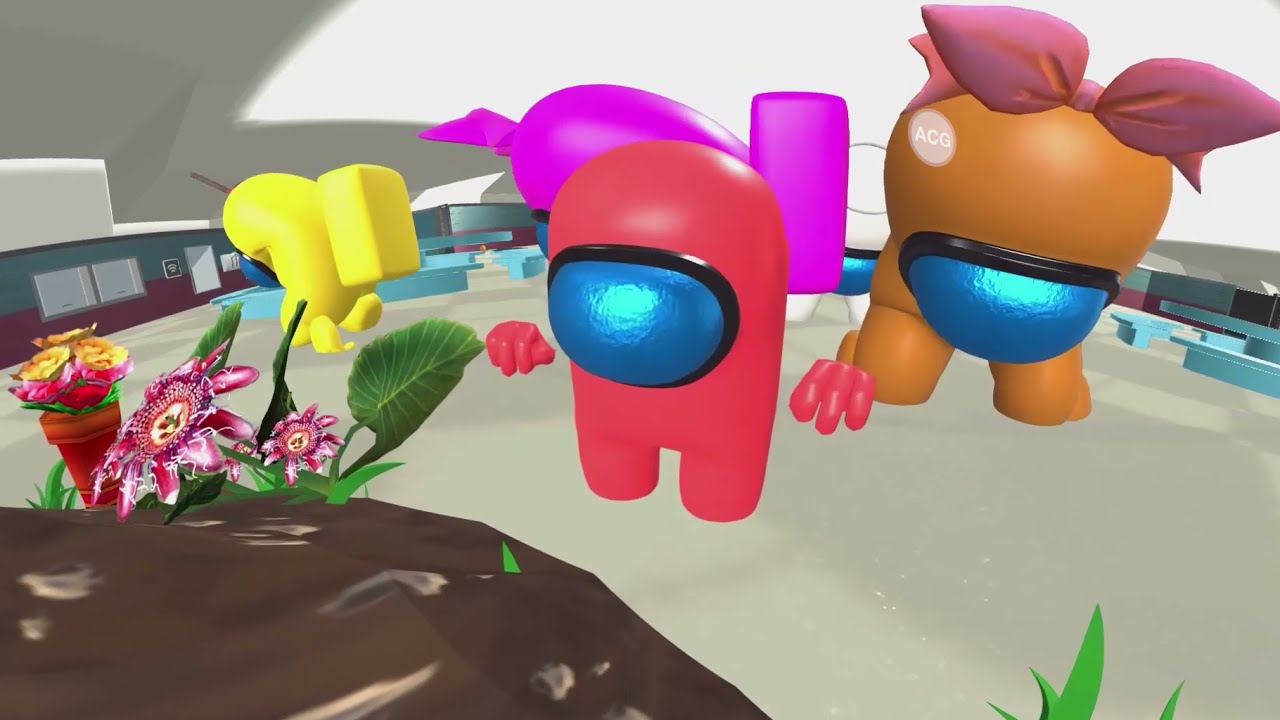The image is a detailed 3D video game screenshot featuring four cylindrical characters with two legs and no visible arms, each identifiable by their distinct colors and accessories. A red character with a blue visor-like "Cyclops eye" stands prominently in the center. To its side, an orange character features a pink bow on its head. Another yellow character, distinguished by a yellow backpack, is also present. Additional details include a fourth character, noted to be purple by one description but missing in others.

The scene takes place inside a large building with gray and white walls and ceiling. The floor is light gray, except for a sandy or rocky patch in the lower left corner adorned with a flower pot containing vibrant yellow, pink, and red flowers, along with another brightly colored flower featuring purple, white, and red hues and green leaves. The overall environment has a detailed 3D look, enhancing the visual appeal of the characters and their surroundings.